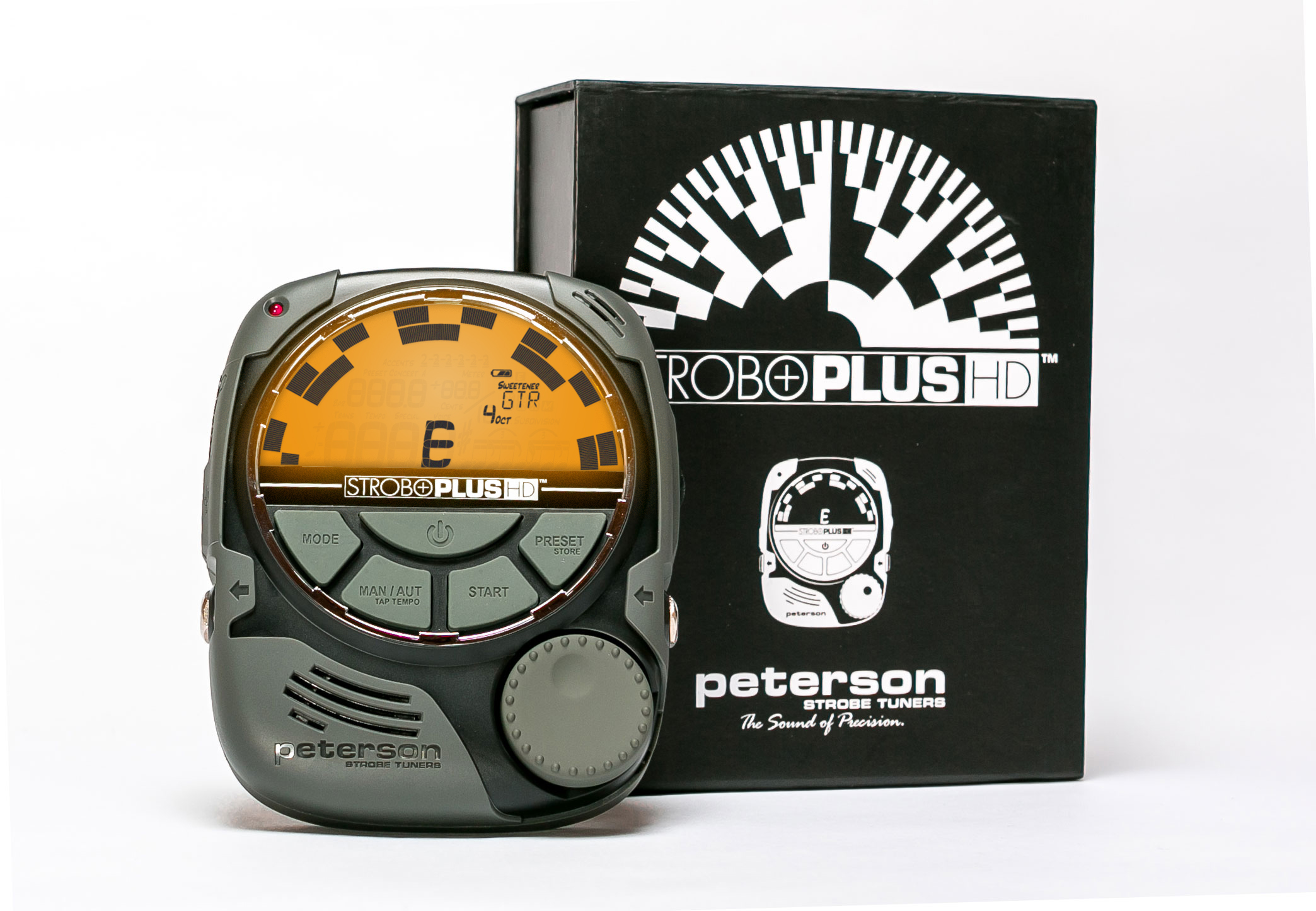The image showcases a Peterson Strobe Tuner product alongside its packaging. On the right side, the black box features white text that reads "Strobo Plus HD," with "HD" in black text on a white background. Above this, there is a semi-circular meter with white and black squares and shapes, resembling steps. Below, it states "Peterson Strobe Tuners, the sound of precision," along with the Peterson logo.

On the left side of the image is the product itself, a gray, almost square device with rounded corners. The device's top has a circular meter displaying the letter "E" in the center. The meter is yellow, marked with one, two, and three bars each side of the center. Below the meter, the device also says "Strobo Plus HD." The interface includes several buttons: Mode, Manual to Auto, Tap Tempo, Start, and Preset, with a central power button. At the bottom right of the device is a tuning dial, and in the bottom left corner, the Peterson logo appears once more. This detailed setup highlights the precision and branding of the Peterson Strobe Tuner.